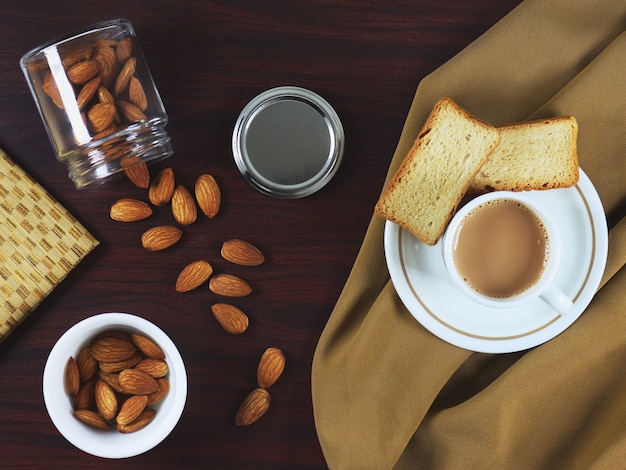This overhead photograph captures a meticulously arranged table setting with a variety of objects and food items. At the top left corner, a clear glass jar lies on its side, its silver lid sitting beside it. The jar, previously filled with almonds still in their brown skins, has spilled its contents onto the dark brown table. Below this, there is a small white bowl also containing almonds. 

In the right-hand section of the image, a tan-colored woven material, possibly a napkin or tablecloth, extends across the table. Positioned on this are a white saucer with a gold rim and a matching white cup filled with coffee. Next to the cup, resting on the same saucer, are two pieces of what appear to be pound cake. 

Adding to the detail, there's a yellow napkin with two shades of lighter and darker yellow rectangles near the small bowl of almonds. The overall composition contrasts the dark surface of the table with the bright, carefully arranged items, creating an inviting and warm tabletop scene.